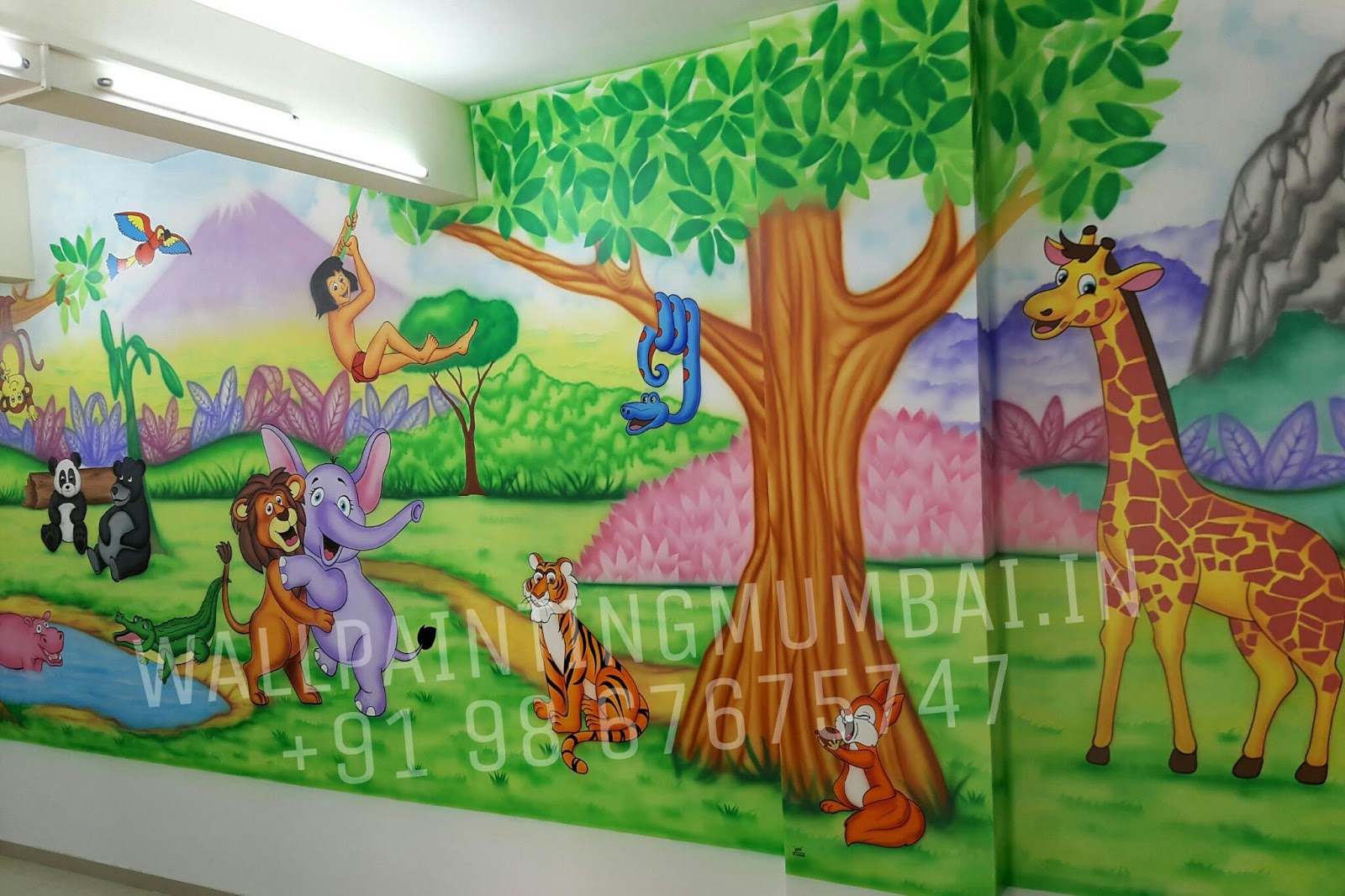This vibrant and vividly colored cartoon-style mural, potentially located in a daycare or school, showcases a lush jungle scene inspired by The Jungle Book and early Disney cartoons. Watermarked with "wallpaintingmumbai.in" followed by the contact number "919867675747" along the bottom, it spans from floor to ceiling, possibly in the corner of a room. Dominating the scene is a large tree at the center, adorned with a smiling blue snake with red dots wrapped around its branches. To the right of the tree stands a cheerful giraffe with happy cartoon eyes, while a friendly squirrel sits at the base. Swinging from a vine on the tree's left side is a young boy reminiscent of Mowgli. Below him, an elephant and a lion embrace. In the nearby pond, a hippo is partially submerged with a crocodile at its edge. The background features a panda and a grey bear beneath a brightly colored macaw in flight. Amidst the lush greenery and vibrant flowers, a regally posed tiger sits near the tree. A scenic mountain range provides a stunning backdrop, enhancing the mural's sense of depth and wonder.